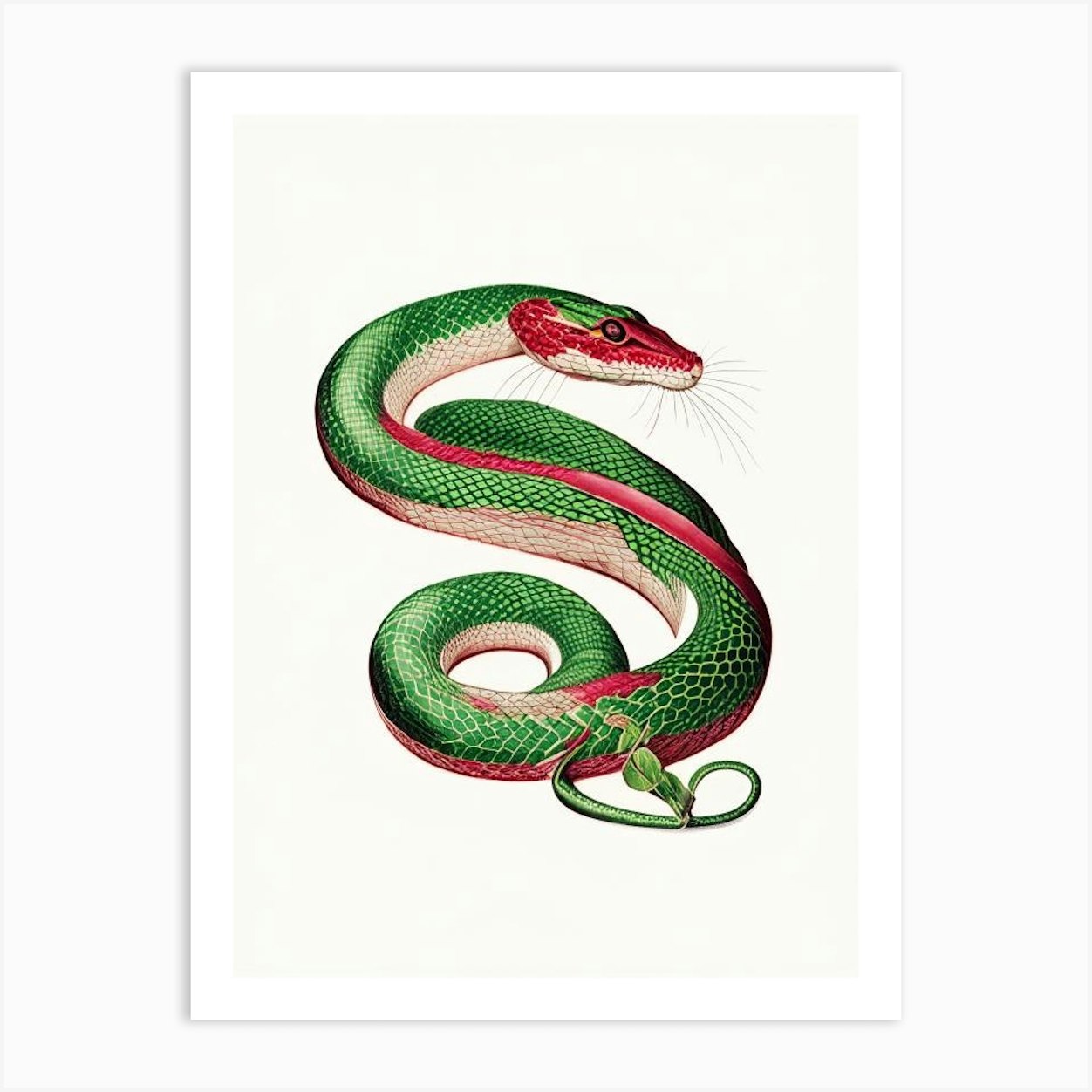This is a detailed drawing of a green and red snake prominently featuring a striking blend of colors and intricate details. The image is set against a backdrop with a white and light gray border. In the center, the snake is depicted in an elegant S-shaped curve, creating a dynamic composition. The head of the snake, located at the top of the picture, is distinguished by its red color, transitioning into white underneath, with a pair of black eyes adding a sense of alertness. The green color starts above the red on his head and continues down the top half of his body, turning into white halfway down his length. Notably, a band of pink meanders around his scaly, green and white body, adding to the visual complexity. 

The snake's mouth is closed, projecting an intense and focused demeanor as if poised to strike. Additionally, whisker-like extensions from his head enhance his formidable appearance. At the bottom right of the image, there’s an ambiguous object that looks like a leaf or a flower, contributing an element of mystery. The snake's tail loops around under him, completing the graceful curve. Overall, the drawing captures the essence of the snake's vigilance and fluidity against a minimalist background.